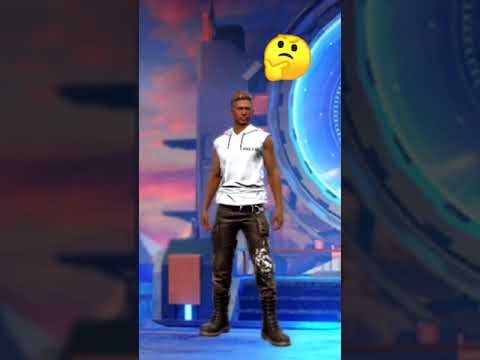In this detailed image, we see a computer-generated character selection screen from a video game featuring a black man in his 30s. He has tan skin and short brown hair, with no facial hair. He is wearing a sleeveless white hoodie, black jeans, a belt, and black camo boots that reach up to his knees. A white design is visible on his left knee. The man is standing in a straightforward stance on a blue floor, with a surreal background that includes a pinkish-blue sky with clouds and a few steps leading up to what looks like a metallic portal with a blue circular center behind him. In the upper right corner of the image, there is a yellow emoji with two black eyes, a contemplative facial expression, and its hand up under its chin. The surroundings also have additional border visuals with darker lighting, framing the central image.